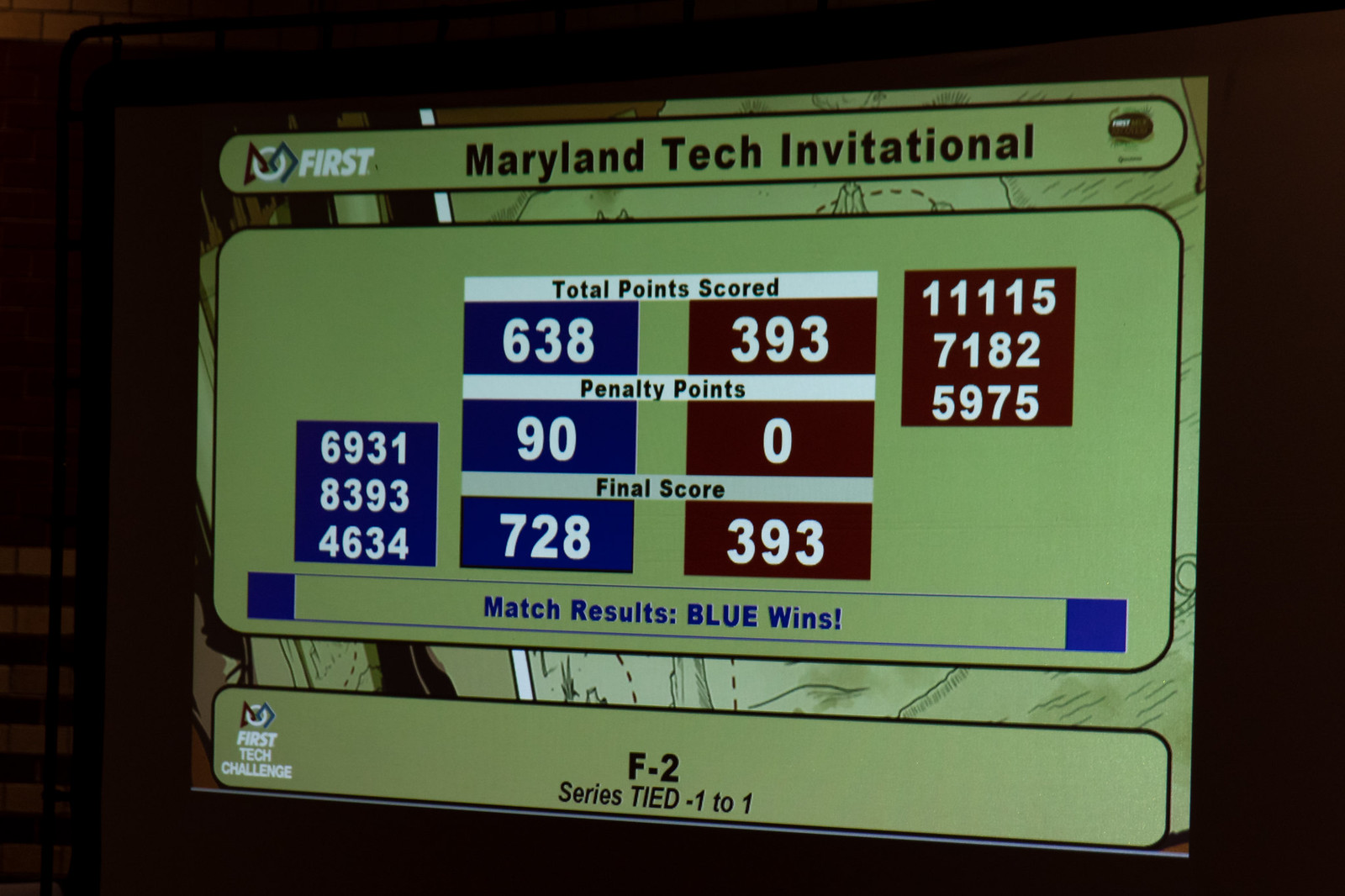This photograph displays a detailed scoreboard from the Maryland Tech Invitational sports game. The scoreboard has a light green background and prominently features the text "Maryland Tech Invitational" at the top. The scores are presented within colored rectangles: blue rectangles for one team and red for the opposing team, with white letters and numbers. 

At the top, under "Total Points Scored," the blue team has 638 points while the red team has 393 points. Below this, "Penalty Points" shows that the blue team conceded 90 points, whereas the red team conceded none. The subsequent section, titled "Final Score," lists the blue team with a score of 728 and the red team with 393. The results at the bottom declare "Match Result: Blue Wins," emphasizing a victory for the blue team. Additional text notes that the "F2 Series is tied 1 to 1." The scoreboard is symmetrically designed with other numbers present in smaller rectangles on either side, although their specific significance isn’t apparent. Overall, the scoreboard offers a comprehensive view of the game's outcome.